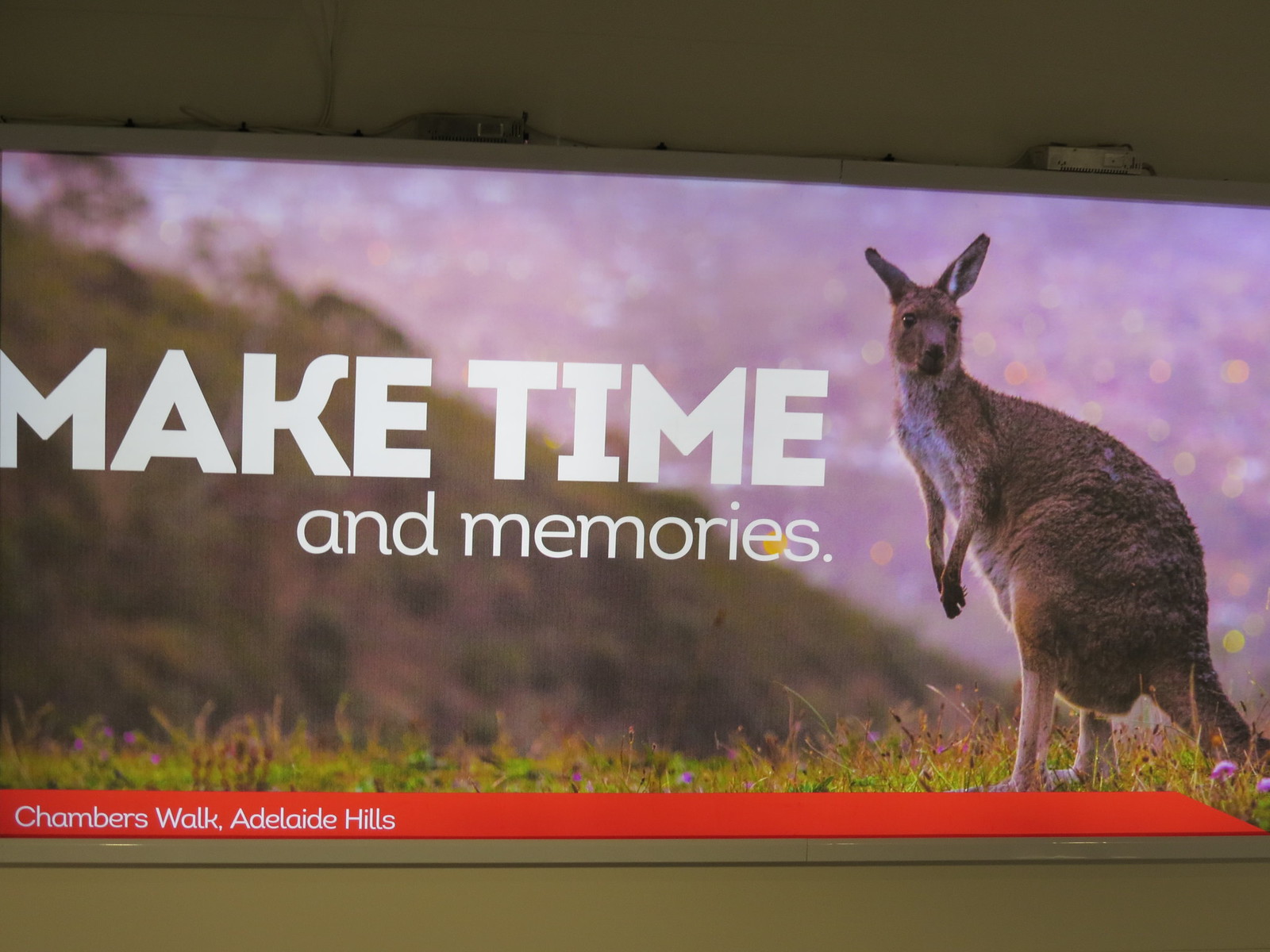The image is a photograph of a poster advertisement, likely seen in a public space such as a subway station or the interior of a car. The poster is set against a greenish-tinted, olive-tan background and features a prominent kangaroo or wallaby standing on a grassy knoll. The animal, with its tan body, white chest, and a small white streak on its right ear, looks directly at the camera. Behind it, there are hills and a blurry cityscape with lights, suggesting twilight transitioning into night. To the left of the kangaroo, the slogan "Make Time and Memories" is written. Beneath the image, in an orange band with white text, it reads "Chambers Walk, Adelaide Hills," inviting viewers to visit this scenic location in Australia.